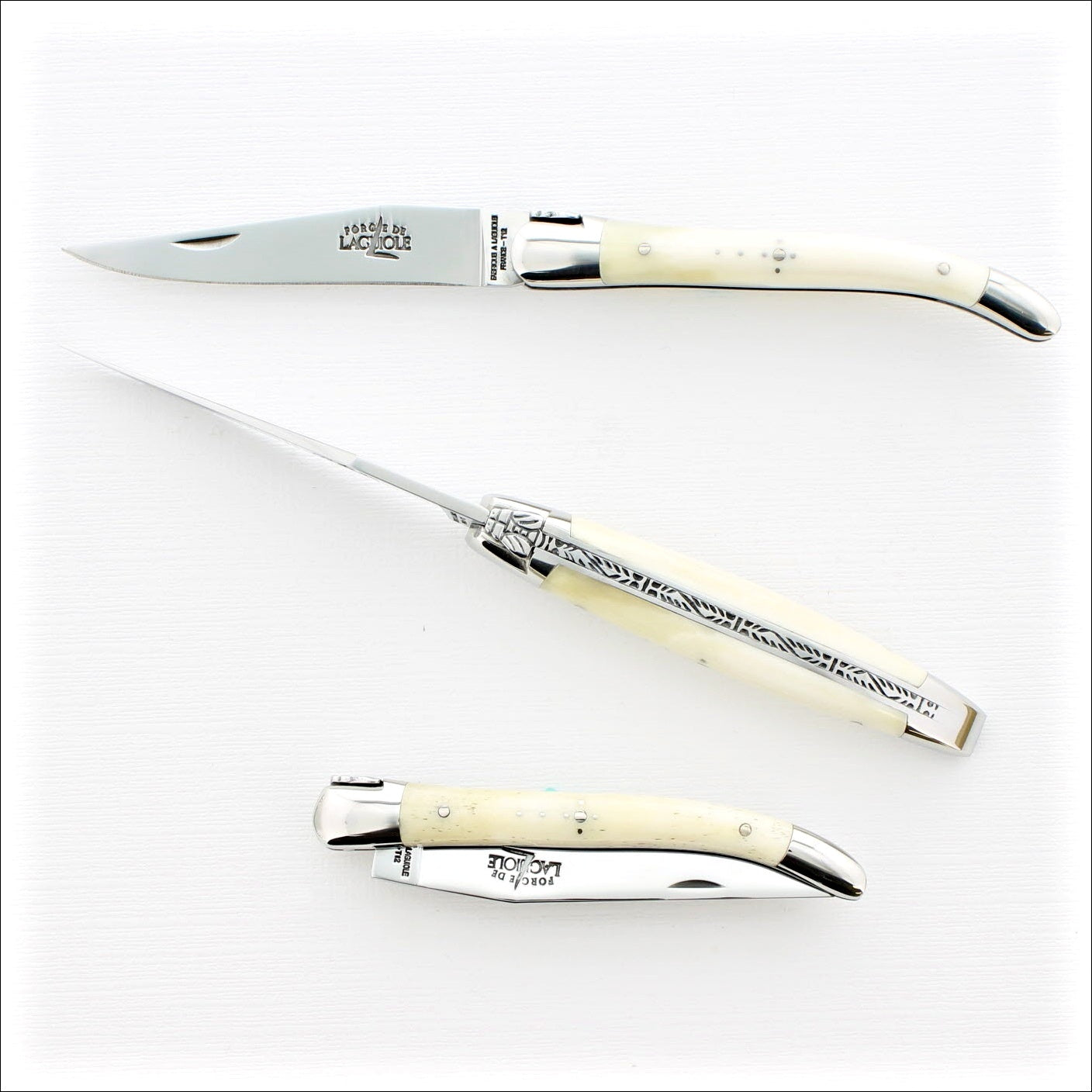This image showcases three pocket knives displayed against a plain white background. The top knife is fully extended, prominently revealing its short, pointed silver blade and sleek white handle that appears to be made of ivory or a stone-like material, accented with three silver dots and silver detailing at both ends. The middle knife is positioned diagonally from the bottom right to the top left corner, lying on its blade, allowing a view of its narrow edge and a decorative metal design with intricate carvings, bearing the inscription "Forge de Laguiole." The bottom knife is completely folded, with the blade tucked neatly into the handle, showcasing the same distinctive white handle with silver embellishments. Together, these views provide a comprehensive depiction of the knife's design and functionality from different angles.